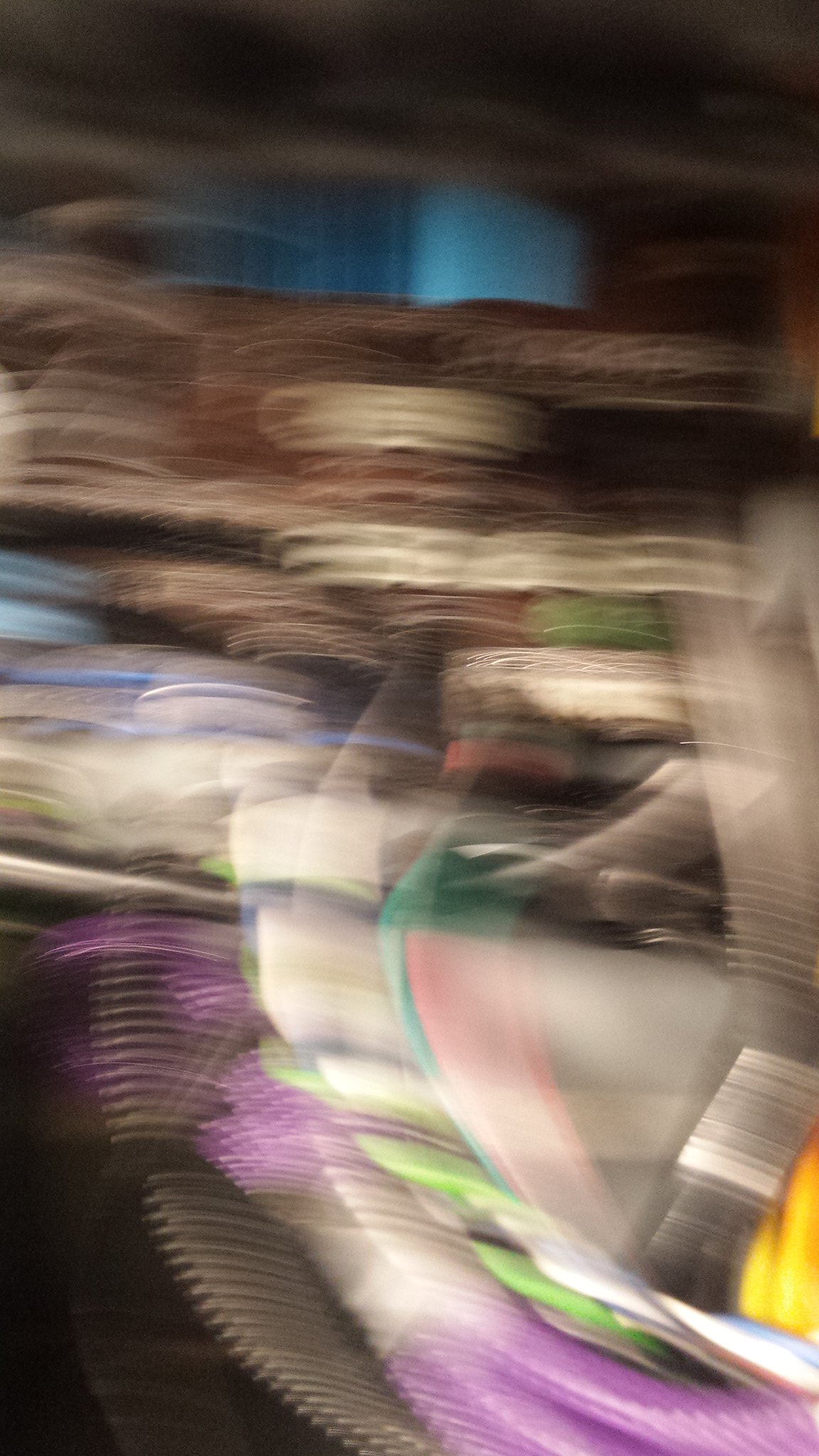A completely blurry photograph presents an abstract composition with no discernible focal point. At the top, an expanse of blue suggests a sky or backdrop, transitioning into a repeating brown and tan pattern that might imply a textured surface or layered object. Beneath this, a section of white merges with shades of blue and hints of teal in the middle, adding to the visual enigma. In the lower right corner, the faint presence of what appears to be a barcode adds a touch of identifiable detail to an otherwise perplexing image. Despite the lack of clarity, the varied colors and vague patterns invite curiosity and multiple interpretations.